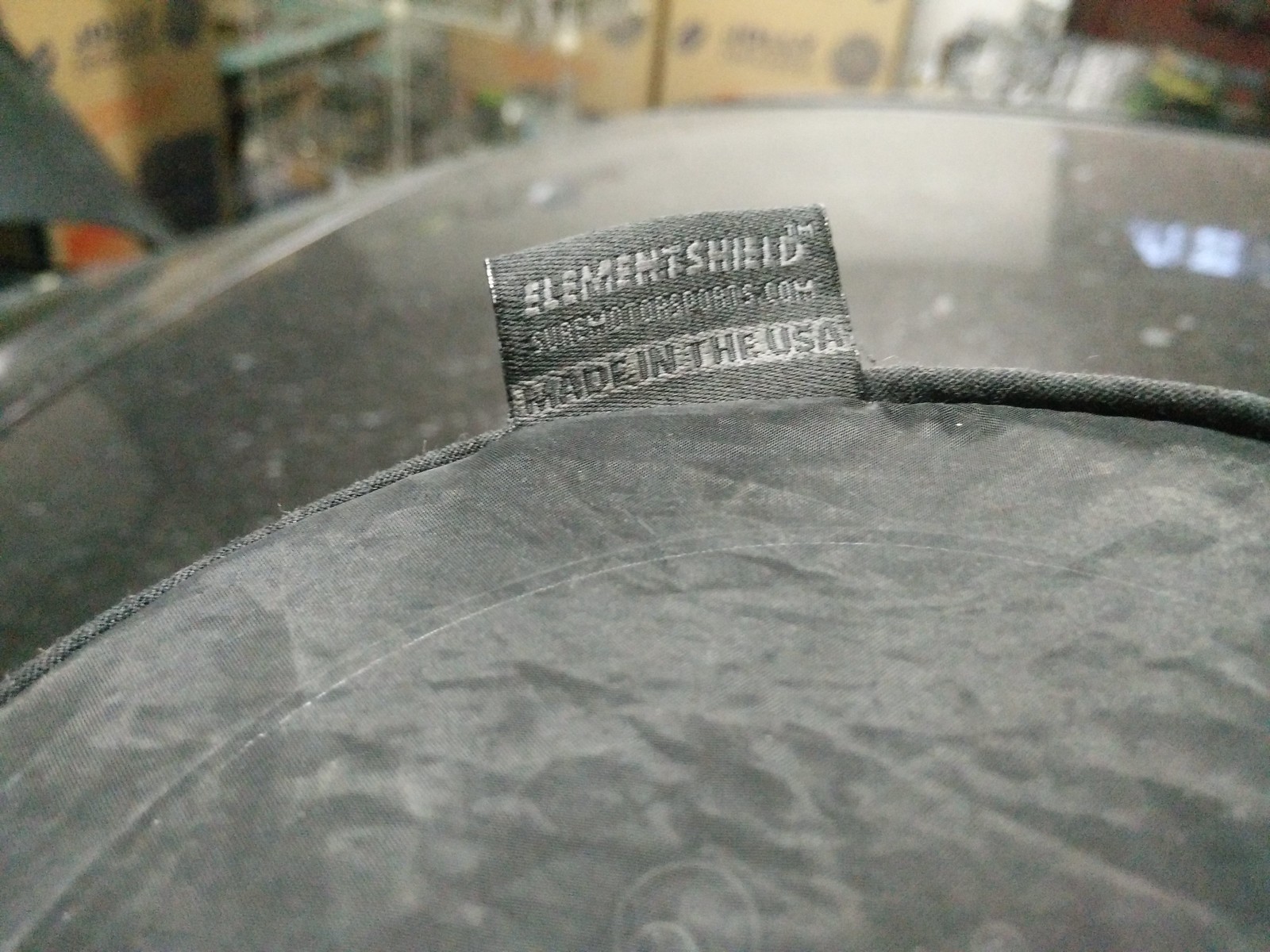In this image, taken possibly in a department store, we see an extreme close-up of a gray circular cloth item in the foreground. Sticking up from the cloth is a tag in the shape of a rectangle. The tag has a gradient of light to dark gray and prominently features the words "Element Shield" in white font, with a TM (trademark) symbol at the top right corner of the 'D.' Below this, in smaller white font, it reads "Shore Motorsports.com." At the bottom of the tag, a thin white line extends horizontally, enclosing the phrase "Made in the USA" in gray lettering. The background is somewhat blurry but gives a hint of a brown wall and possibly a clear section which might be part of the shield itself. The setting suggests the store could be related to sports or camping equipment.